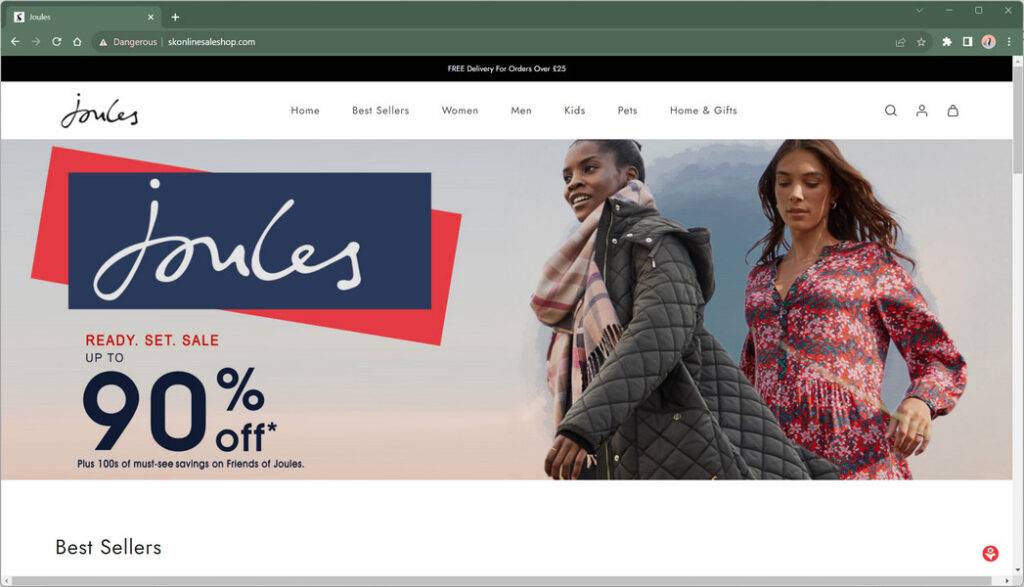In the image, the top section features a darker green header on a computer screen with an inaccessible tab. Below this, there's an unreadable website name, followed by a black bar that offers a free delivery promotion, though the specific details can't be discerned. The primary website shown is "Joules" (spelled J-O-U-L-E-S) on a white background. Across the top, horizontally listed are navigation options: Home, Bestsellers, Women, Men, Kids, Pets, Home and Gifts, along with three icons (search, user, and a folder-like symbol).

In the middle section of the website, there's a gradient background transitioning from dark tan to blue. The company's logo, "Joules," is prominently displayed on a dark blue background with a red accent behind it. “Joules” is written in white text. To the right of the logo are images of a black woman and a white woman. Below the logo, there's a promotional message: "Ready, Set, Sail - Up to 90% Off," with additional terms and conditions listed underneath.